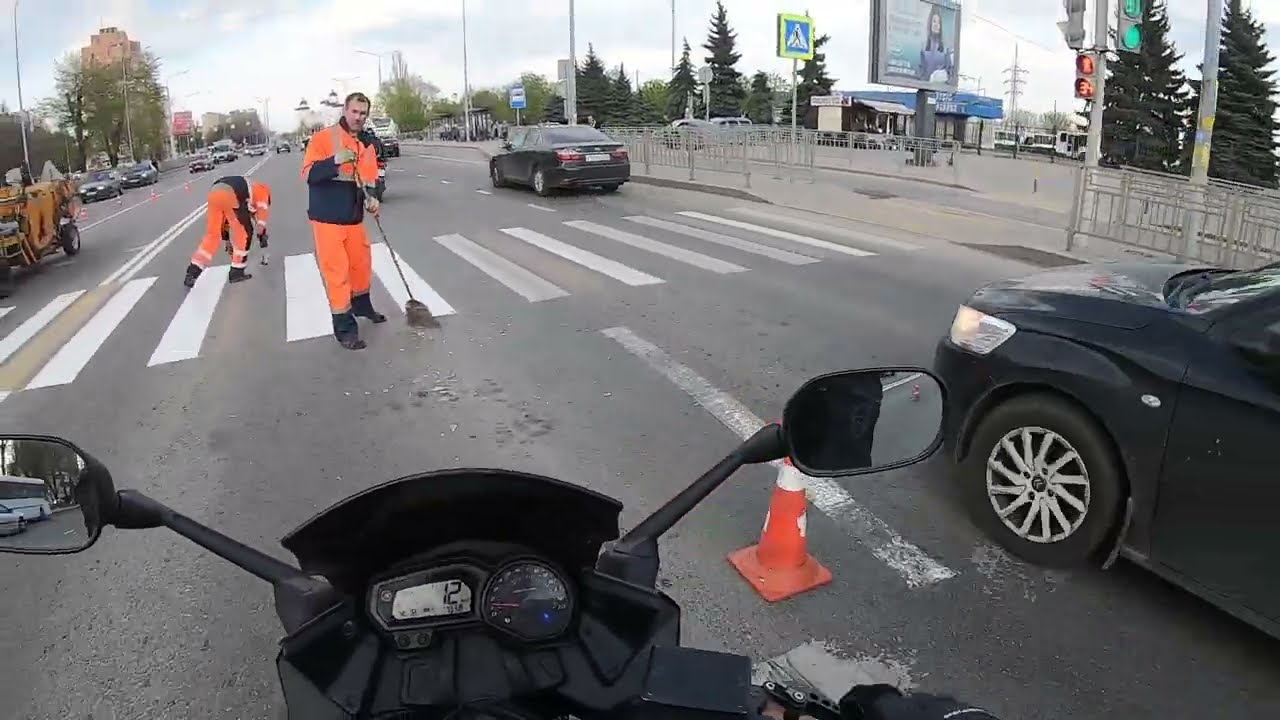In this urban street scene, the photograph captures a pedestrian crossing from the viewpoint of a motorcycle rider on a black bike, positioned in the middle of a three-lane road. On the pedestrian crossing ahead, two men in orange and black uniforms are at work: one man is sweeping the ground, while another is bent over, picking up debris. To the right of the motorcycle and at the front of the crosswalk, a black vehicle is parked, accompanied by an orange traffic cone. In the background, various vehicles travel along the opposite three lanes, with a yellow utility truck and additional orange cones visible. The sky overhead is clear with blue hues and scattered white clouds. The scene includes billboards, traffic lights, poles, trees, and some nearby businesses, further emphasizing the urban environment.